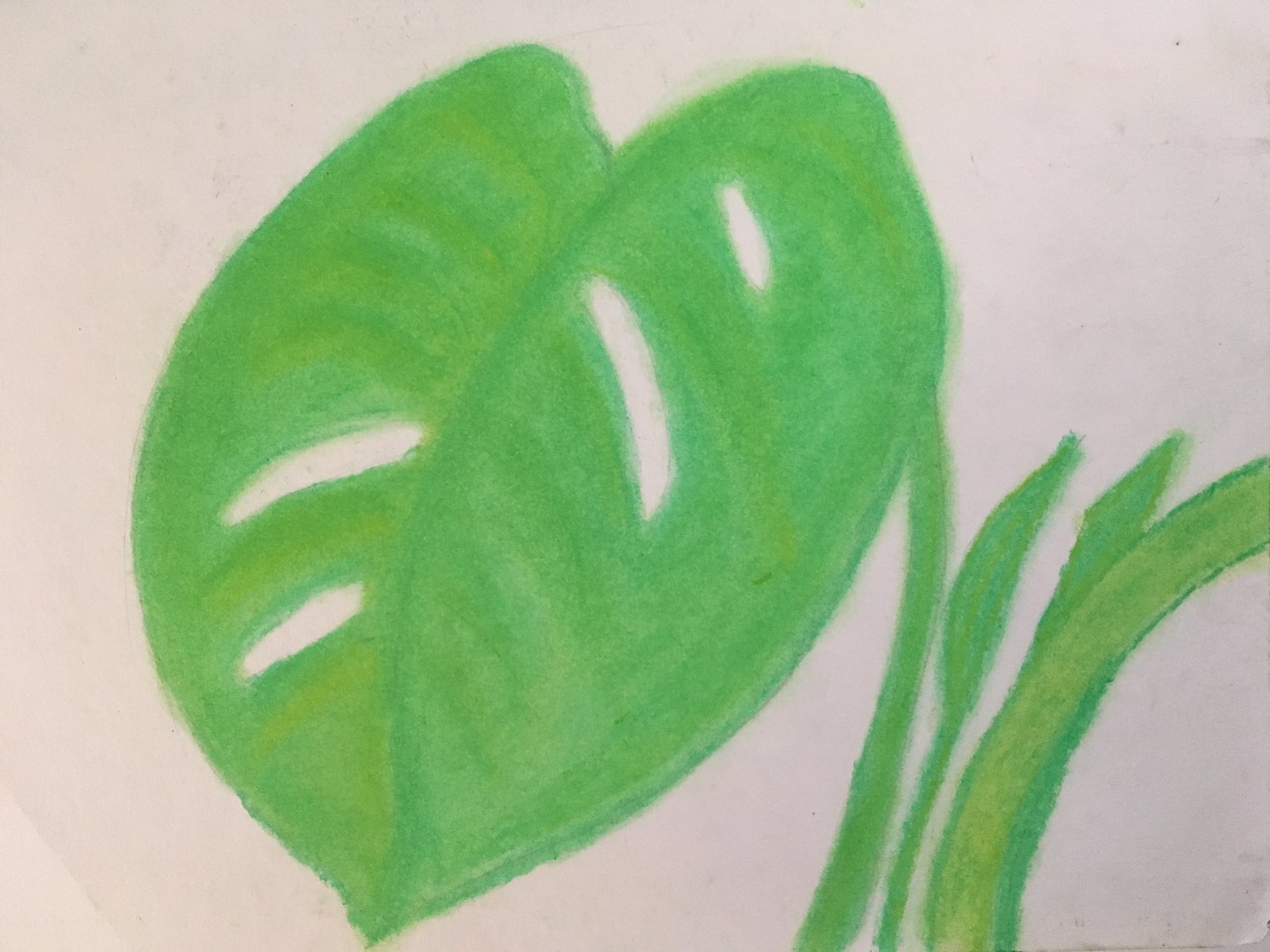A beautifully detailed crayon sketch showcases a large green leaf, characterized by a prominent central fold and carefully drawn veining. The leaf features distinct slits or reflective shine marks, enhancing its realistic appearance. The soft, slightly faded edges of the leaf blend seamlessly into the off-white background of the sketch pad. Adjacent to the main leaf, vertical reeds and longer leaves, colored in various shades of green, add depth and context to the composition. This captivating illustration combines artistic simplicity with intricate details, highlighting the leaf's natural beauty and the surrounding greenery.